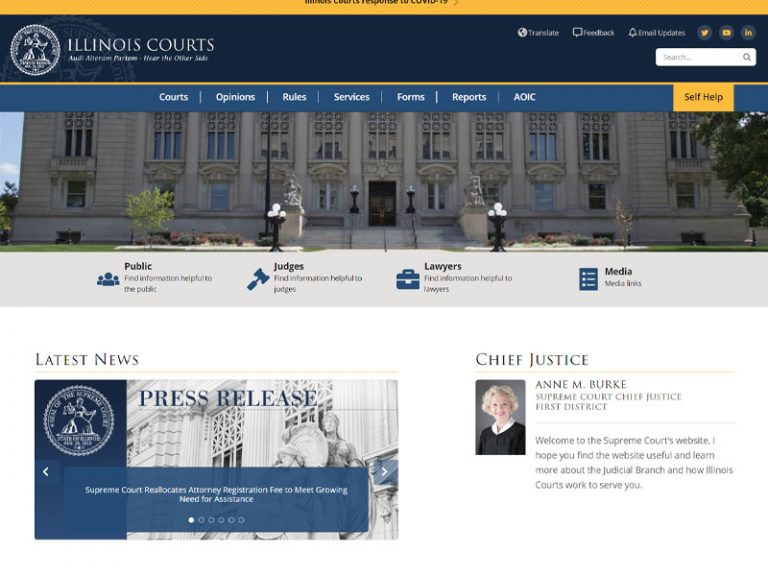The image features a distinct orange border at the top followed by a navy blue header. On the left side, there's an official-looking circular seal, likely representing the Illinois courts. Adjacent to the seal, there's text that reads "Illinois Courts." Social media icons for Twitter and Instagram are present at the top.

Below this section, there's a search box. Underneath the search box, there is a grayish-blue navigation bar that includes clickable options such as "Court Opinion," "Rules," "Services," "Forms," and "Report." Next to an orange box labeled "Self-Help," there's an image of a stately building with columns in the front and statues that appear to be lions.

Further down, there's a gray bar listing options such as "Public," "Judges," "Lawyer," and "Media," followed by a "Latest News" section.